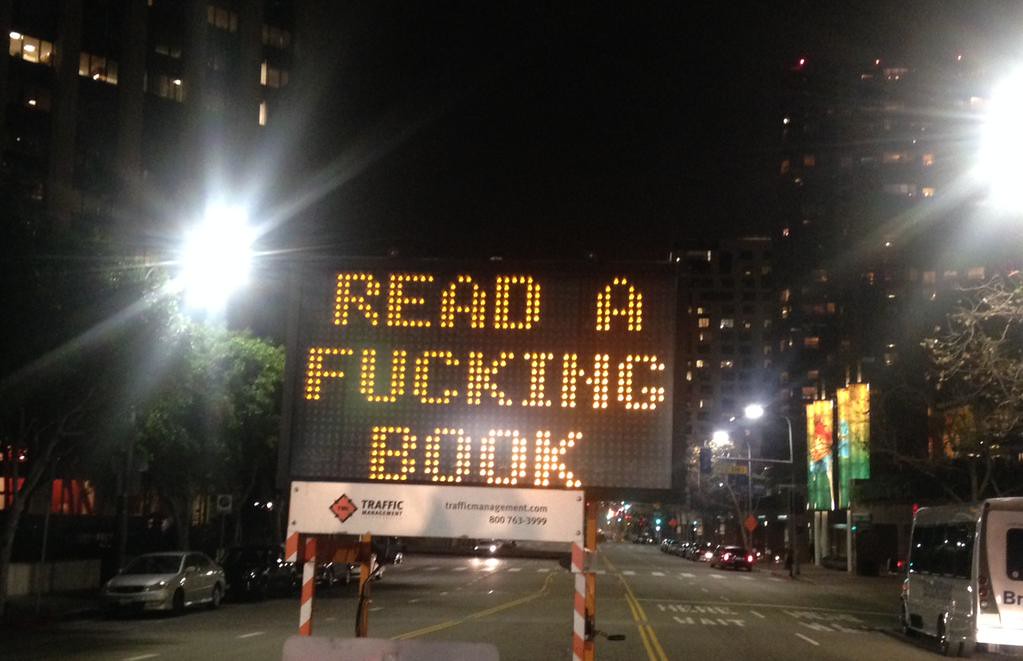The image is a night scene set in what appears to be a downtown area, with tall buildings, some resembling skyscrapers or business buildings, in the background. The dark night sky contrasts with the various lit windows, casting a yellowish hue. The street in the foreground is busy, lined with parked cars on both sides, featuring colors like white, black, and silver. Streetlights, both on the left and right, illuminate the scene, creating a flashy ambiance.

In the center of the image, dominating the road, stands a digital traffic sign set on a black platform with orange and white striped legs. The sign prominently displays the message "READ A FUCKING BOOK" in vivid yellow lights. This sign rests on black asphalt marked with yellow stripes and a white crosswalk.

Adding to the urban clutter, there are hoardings and green trees on both sides of the street, along with flags in shades of yellow, orange, and green fluttering along the sidewalks. A blue and black van is parked on the right side of the road, contributing to the array of colors captured in the image. The overall scene is drenched in artificial light, typical of a bustling city at night.